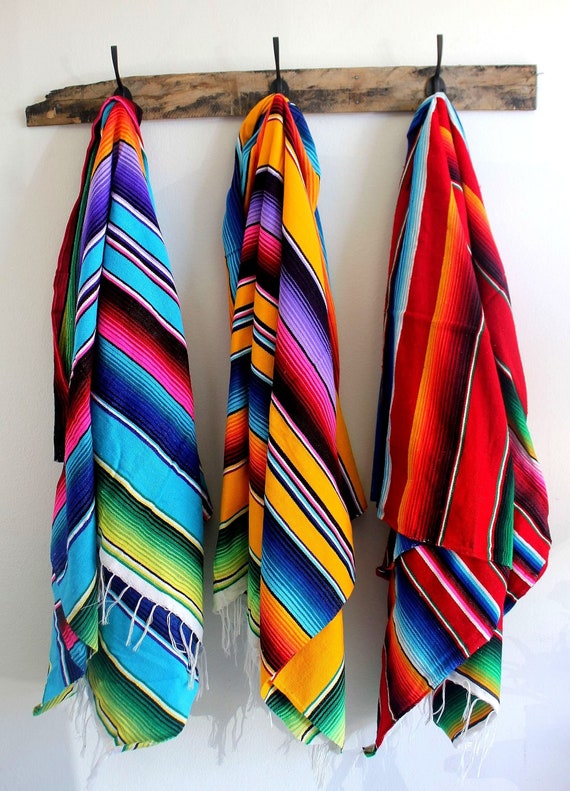This photograph captures a detailed scene featuring three vibrant, multicolored scarves hanging on a rustic wall-mounted rack. The rack itself is crafted from a piece of weathered, brownish wood with black blemishes, giving it a somewhat antique and textured appearance. Attached to this wooden strip are three U-shaped black hooks, each holding a scarf.

The scarves are characterized by their dynamic color schemes and striped patterns with vivid hues that vary across each piece. The one on the left predominantly features light blue, interspersed with dark blue, black, hot pink, red, green, and purple. This scarf also has wide and thin stripes and is finished with a white fringed hem.

The middle scarf displays a palette dominated by yellow and purple, accented with black, white, red, hot pink, various shades of blue, and green at the bottom. Its design is consistent with the first scarf, with alternating vibrant and black stripes and a similar white fringe at the bottom.

The rightmost scarf showcases a striking combination of red, orange, black, white, blue, and green, following the same general design theme. It too is finished with the characteristic white fringe.

The backdrop of the scene is a plain white wall, which highlights the scars’ lively colors and intricate stripe patterns. The overall composition is clear and focused, with the vivid colors casting subtle shadows on the wall, adding depth to the image. There are no other elements such as text, people, animals, or plants within the frame, keeping the viewer's attention solely on the displayed scarves.